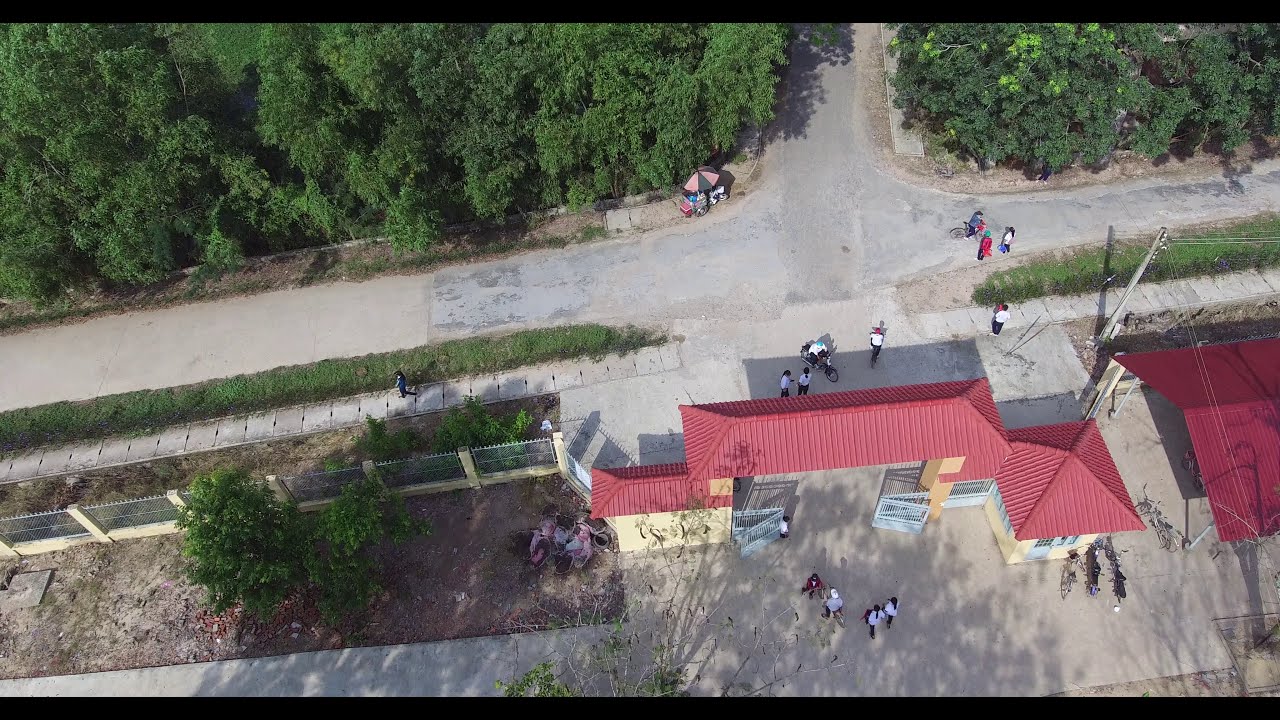This high-angle drone photograph captures the bustling entrance of a tourist attraction or historical site. The focal point is a prominent red-tiled roof gateway, supported by two pillars and featuring a double-wide gate that stands open, inviting the steady flow of visitors. People on foot and bicycles are seen moving in and out, traversing a mix of paved and gravel paths that extend beyond the gate. On the corner of the entrance, a street vendor with a distinct pink and gray umbrella is selling refreshments, adding to the lively ambiance. The scene is framed by abundant vegetation and forested areas, hinting at the lush surroundings within the gated area. This entrance leads to a large concrete space where more visitors are visible, reinforcing the site's significance as a popular public or tourist destination. The well-maintained sidewalks and asphalt roads inside further denote a frequented location, possibly a park, garden, or historical temple, though no specific landmarks are present to confirm the exact nature of the site.